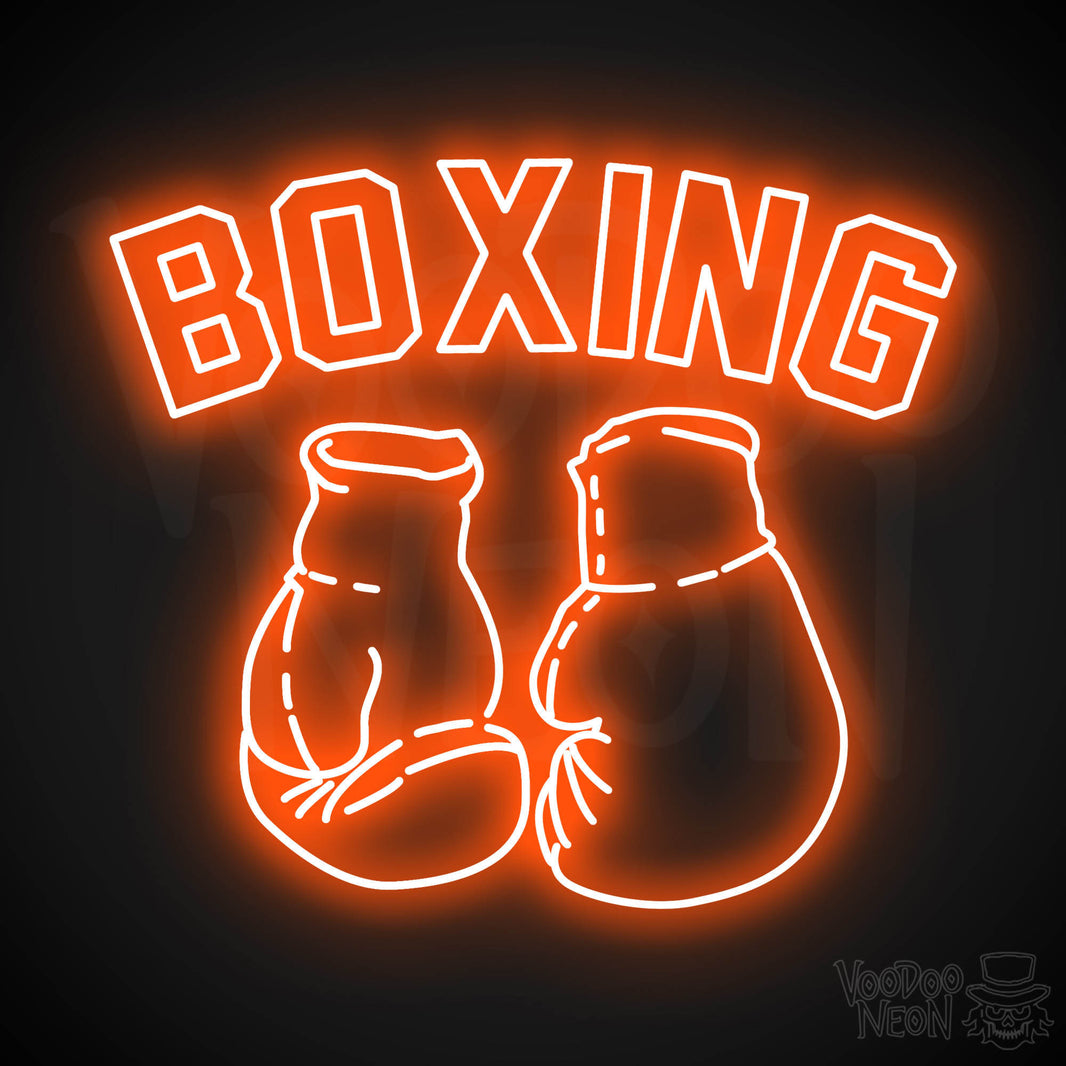The image showcases a vibrant color computer graphic depicting a neon sign with the word "BOXING" and an outline of two boxing gloves. The text "BOXING" is rendered in capital, block-style letters, primarily in white, with a glowing orange-red effect as if made from neon light tubes. This creates a radiant, illuminated look against a dark off-black background. The word "BOXING" arcs gently near the top of the image, with a red drop shadow enhancing its neon effect.

Beneath the text, centrally positioned, are two boxing gloves. The gloves are outlined in the same white and orange glow as the text, adding to the neon light effect. The glove on the left displays its palm towards the viewer, while the glove on the right faces away. Their cuffs extend upwards, almost reaching the word "BOXING" above them.

In the bottom right corner, the image features a small logo with the text "Voodoo Neon" in white. Next to the text is a character's face, resembling a skull or monster with a top hat, adding a unique, somewhat eerie touch to the graphic. The backdrop remains consistently black, emphasizing the neon glow of the main elements.